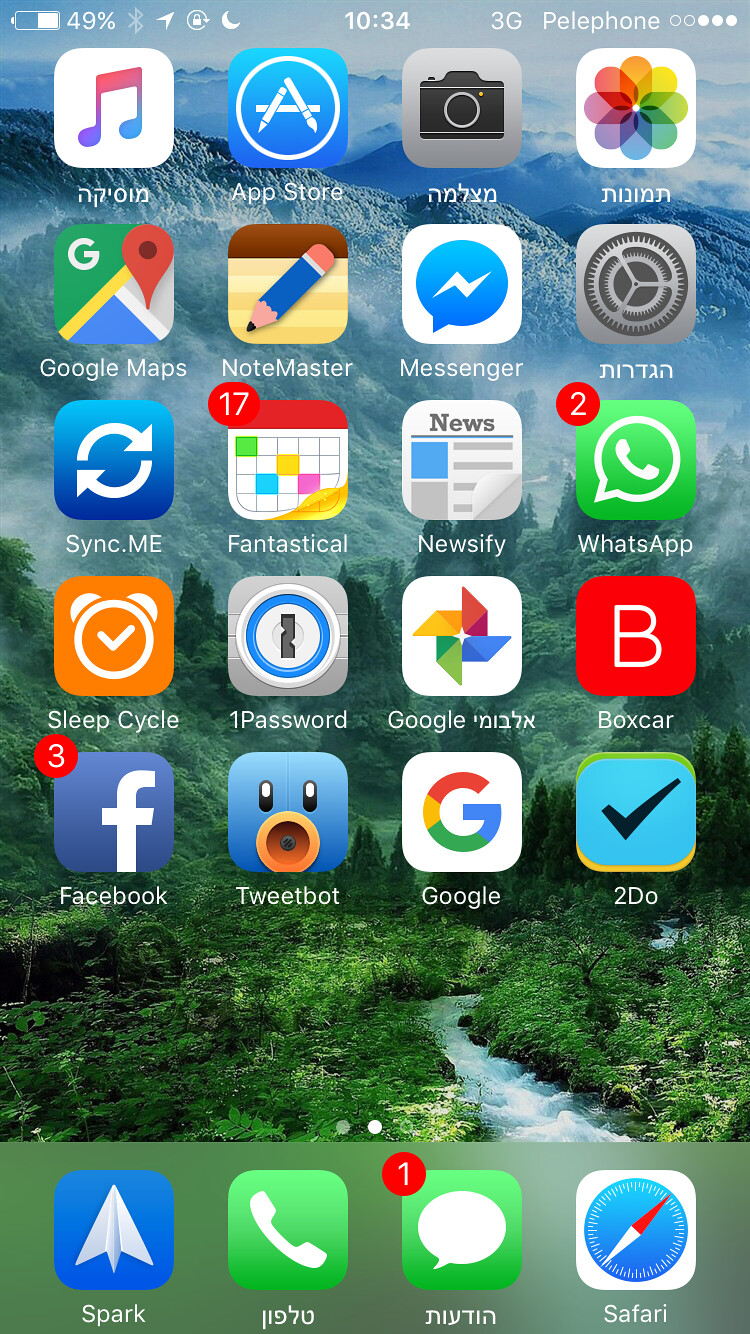The screenshot displays the homepage of an iPhone adorned with a lush, green forest wallpaper featuring a serene stream and a towering, verdant mountain landscape in the background, with clouds settled near the peak. Prominently showcased on the screen are various popular apps, including Google Maps, Facebook, WhatsApp, Messenger, the App Store, iTunes, Preferences, and Notemasters. The app icons are primarily labeled in English, but the interface also includes text in an East Asian language, possibly Indic. At the top of the screen, standard status indicators are visible, showing the battery level, current time, Wi-Fi and Bluetooth connectivity, and additional icons for hibernation and phone lock.